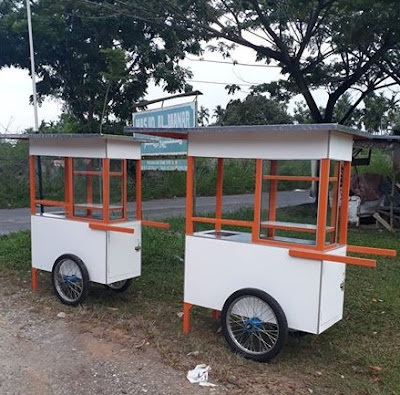In this image, the main focal point is two white, wooden push carts positioned diagonally from one another, mostly centered towards the bottom. Both carts have brown wood accents, including their push rails, stilts, and the railings that support the covers. The covers are white with bold-looking edges. Each cart is equipped with two tires. The scene takes place outdoors, possibly in a Spanish-speaking country, indicated by a sign in a different language, typical of settings where food carts are common. The carts are currently resting on a grassy area beside a street, with a stand and two tall trees visible in the background. The dominant colors in the image include green, white, light blue, orange, brown, and gray. The image conveys a serene moment of these usually bustling carts, reminiscent of scenes where vendors push carts through streets, now momentarily at rest.